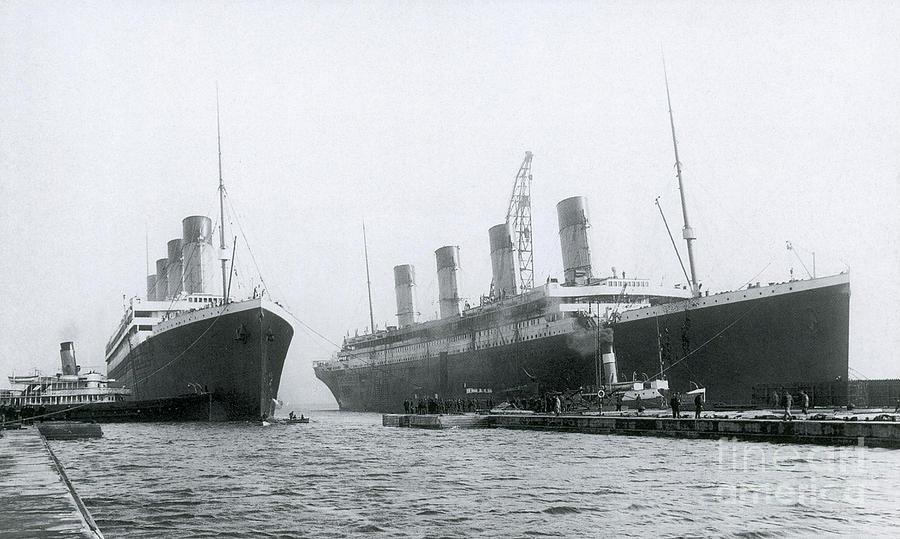A striking black and white photograph captures an outdoor maritime scene in landscape orientation, featuring two massive ships steadily approaching the viewer. The ship on the right is angled more in profile, tilting slightly to the right, while the ship on the left presents predominantly a frontal view. Each ship is equipped with four towering cylindrical structures jutting upward, complemented by visible masts adorned with thin ropes and wires. Along the bottom of the image, a faint group of people can be observed standing on what appears to be a dock, although their details are too indistinct to discern gender or attire. Adding to the scene's complexity, a small boat is situated in the water beside the front of the left ship, seemingly occupied by a couple of people. The composition highlights the grandeur of the ships while subtly incorporating human and small-vessel elements.